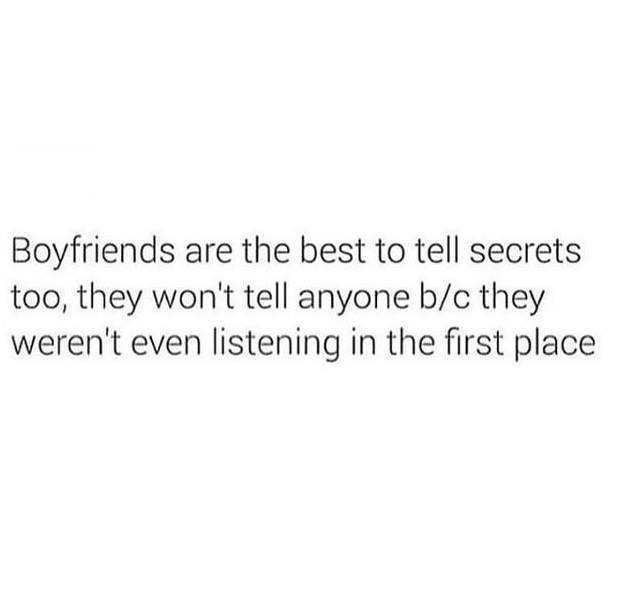The image features a humorous quote on a plain white background, composed using a thin, black Times New Roman font. The quote humorously reads, "Boyfriends are the best to tell secrets to, they won't tell anyone because (B/C) they weren't even listening in the first place." The only capitalized letter in the sentence is "B" in "B/C," which is an abbreviation for "because." The simplistic design lacks any additional imagery or context, focusing solely on the text for comedic effect.